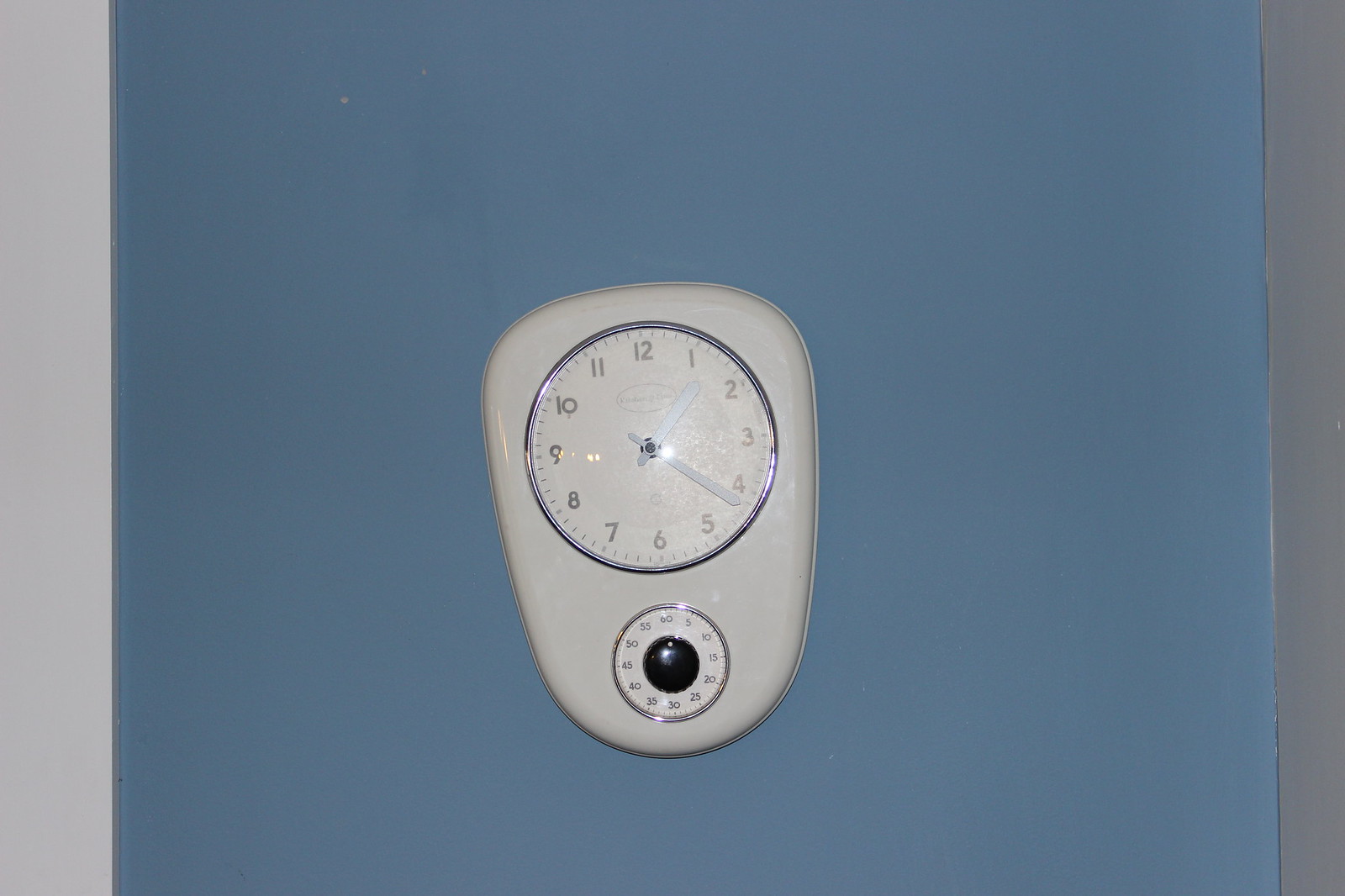The image showcases a clock and thermostat combination unit mounted on a wall. The wall itself features a white trim on the left side and a thin gray trim on the right, with a soft sky blue segment nestled between these trims. At the center of this section is the described clock-thermostat device. The device has a glossy, white ceramic-like exterior with an oval shape that flattens at the top. The bottom portion of this combination unit features a silver circular thermostat with a white face, displaying incremental numbers from 5 to 60 in steps of five and a black middle dial. Above the thermostat, there is a white-faced clock with silver numbers ranging from 1 to 12. The clock hands are positioned to show a time of 1:26.